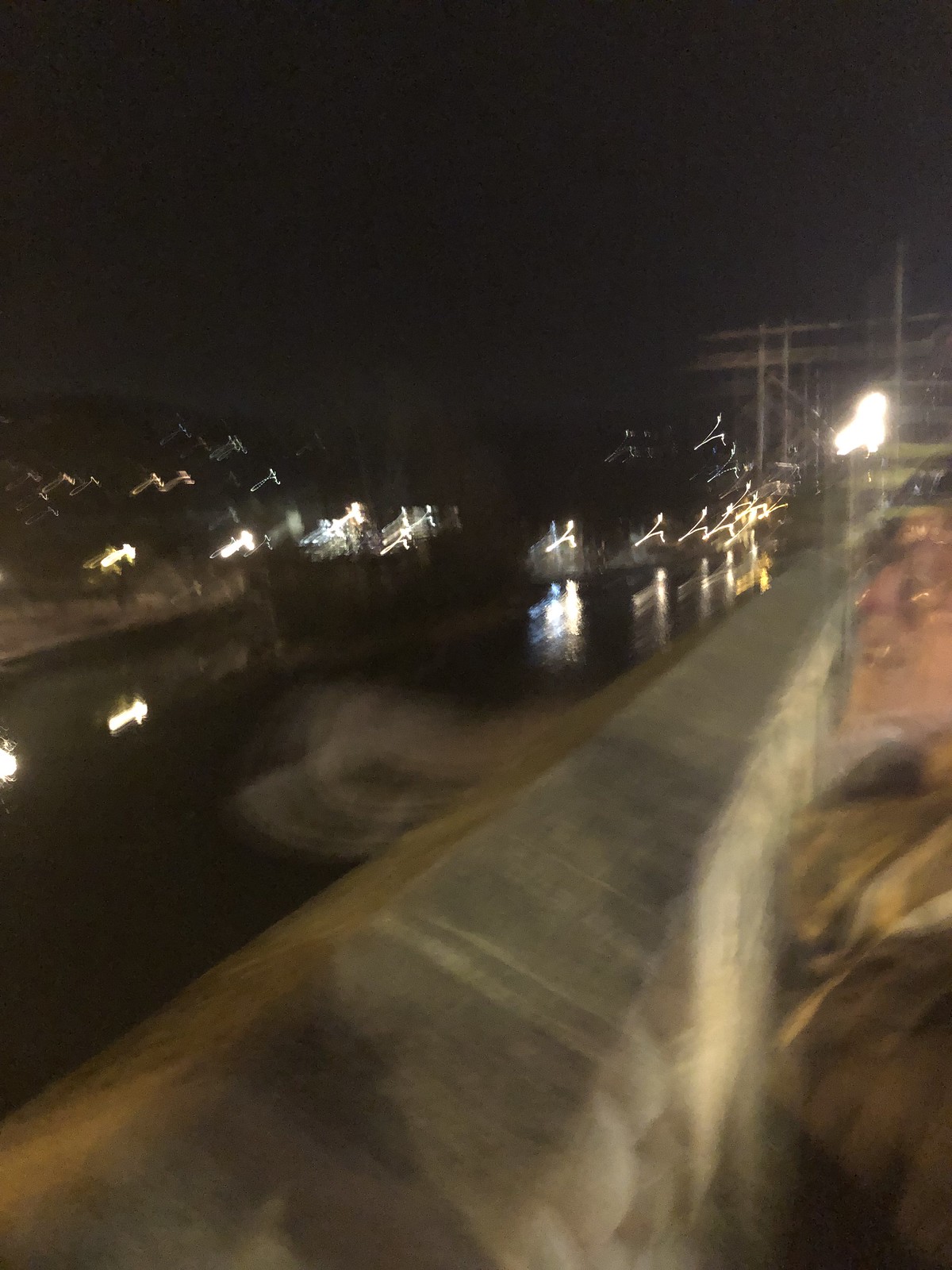In this captivating nighttime image, a group of spectators is seen gathering along a substantial wall at what appears to be a raceway. They eagerly lean over the barrier, their faces illuminated by individual lights they hold, as well as a prominent spotlight casting a bright glow upon them. Below them, a sleek, wet roadway stretches out, its surface glistening under the artificial lights. A procession of cars speeds down the track, their headlights cutting through the darkness.

The thick wall behind which the spectators stand provides a sense of safety and separation from the high-speed action unfolding before them. In the distance, the dim outline of scaffolding emerges, likely serving as grandstands for other onlookers keen to witness the thrilling event. Scattered lights shimmer beyond the racing cars, though their exact nature remains ambiguous. The sky overhead is an impenetrable black, further highlighting the stark contrast between the illuminated raceway and the surrounding night.